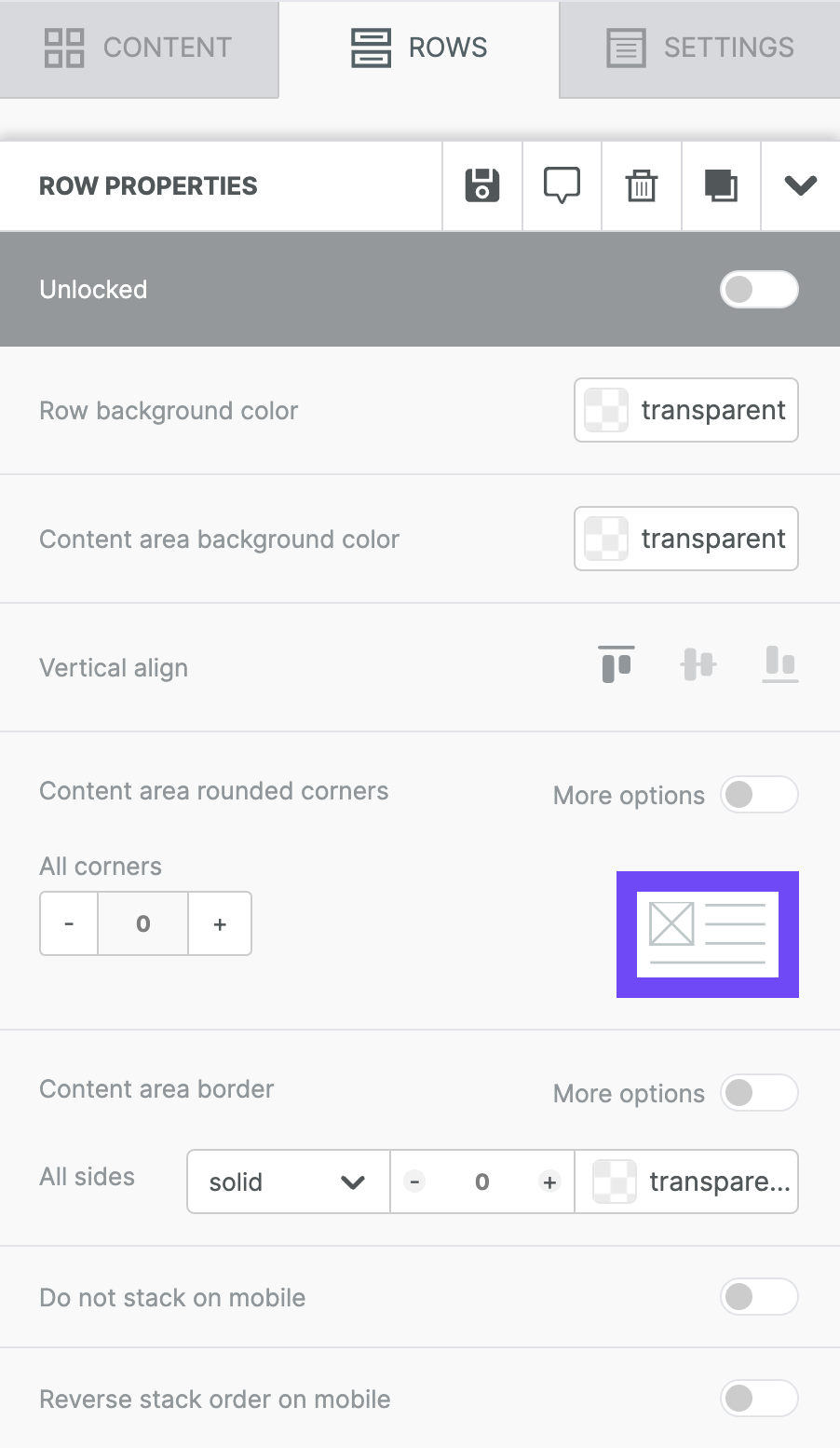This image is a screenshot of a photo editing software interface, possibly Adobe Photoshop or a similar application, captured on a mobile device or tablet. The screenshot showcases the 'Rows' tab, which is one of three tabs located at the top of the page. The other two tabs are labeled 'Content,' represented by an icon with four squares, and 'Settings,' which bears an icon resembling either a piece of paper with text or a cardboard box with a lid.

In the 'Rows' tab, two horizontal rectangles are depicted, each with a line inside, indicating different row properties. Below this section, various controls are available, including a 'Save' button, a 'Message' button, a 'Trash' button, a 'Layers' button, and a drop-down menu button. Additionally, there's an 'Unlocked' toggle option set to 'Off.'

Further customization options are detailed below this toolbar:
- Row Background Color
- Content Area Background Color
- Content Area Rounded Corners
- Content Area Border (All Sides)
- Do Not Stack on Mobile
- Reverse Stack Order on Mobile

This comprehensive set of tools and settings provides users with the ability to finely tailor their editing projects directly from their mobile devices.